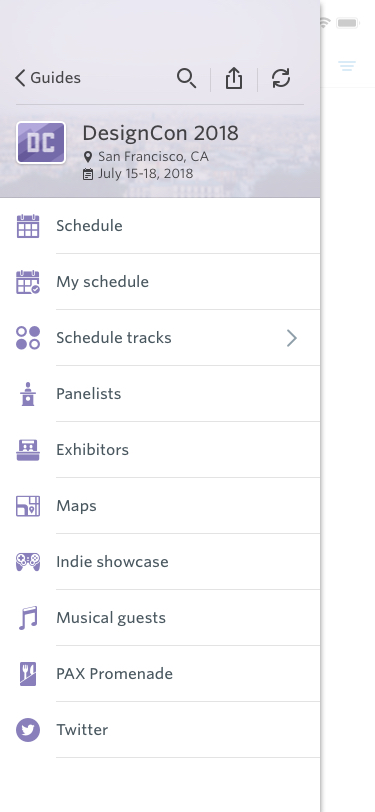This image is a screenshot of an app designed for the Design Con 2018 event, held in San Francisco, California from July 15th to 18th, 2018. The app's interface features a "Guides" section prominently displayed at the top left, alongside the "DC" logo, representing Design Con. Below this branding, the event details are specified clearly. 

The app offers a variety of navigational links to help users access different sections related to the convention. These links include "Schedule," "My Schedule," "Schedule Tracks," "Panelists," "Exhibitors," "Maps," "Indie Showcase," "Music Guests," "Musical Guests," "PAX," "Promenade," and "Twitter," providing comprehensive information and easy access to various segments of the event. 

At the top right of the interface, there are icons for a magnifying glass (indicating a search function), a share or download button, and a refresh button, likely used for updating content such as notifications.